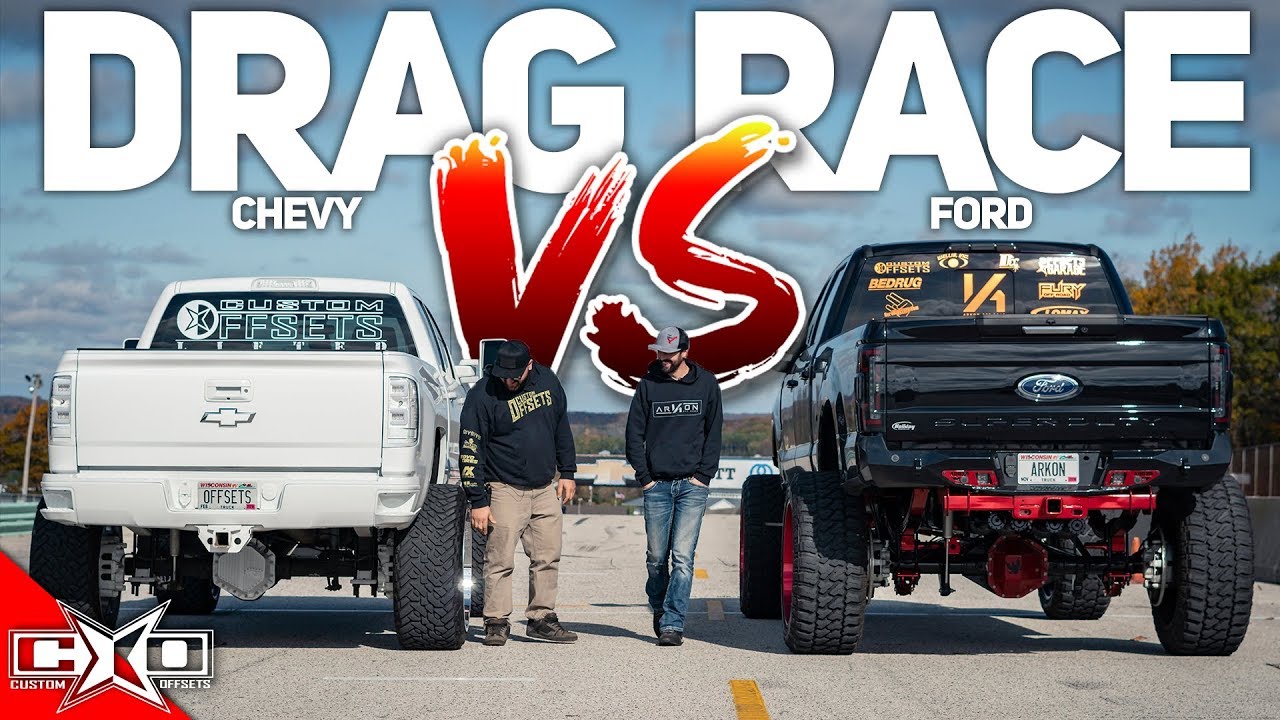**The Drag Race: Chevy vs. Ford**

In this wide image, two towering pickup trucks—a white Chevy on the left and a black Ford on the right—are parked side-by-side in a gray parking lot with precisely marked yellow lines. Above the scene, bold white text reads "The Drag Race," with "Chevy vs. Ford" displayed underneath. This phrase is graphically enriched in the center with the words "versus vs." in a gradient of red, yellow, and maroon, outlined in white.

Both trucks, equipped with massive off-roading tires and lift kits, hint at their formidable performance capabilities. Standing between them are two men, facing the prospective race scene. The man on the left, next to the Chevy, is dressed in a black hoodie, brown khaki pants, and a black hat, while the man on the right, beside the Ford, sports a black hoodie, blue jeans, and a gray cap.

The setting is illuminated by a clear blue sky overhead, and a small red triangle logo in the lower left corner catches the eye. This logo reads "CXO," followed by "Custom Offsets," rounding out the detailed and competitive atmosphere depicted in the image. Notably, the license plate on the Chevy reads "Offsides," and the Ford’s plate says "Accra," adding a personal touch to each vehicle.